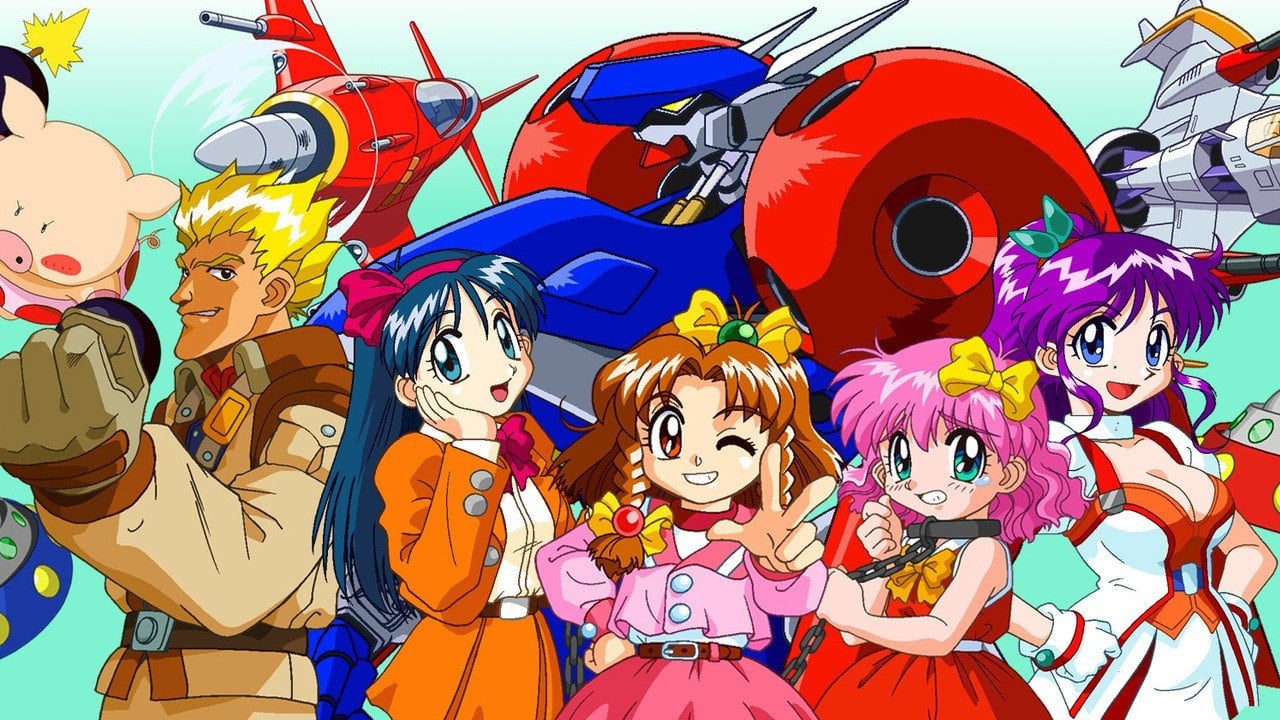In this detailed anime illustration, four distinct anime girls take center stage against a light blue digital background. From left to right, the first girl has long black hair adorned with a bow, big blue eyes, and an almost nonexistent nose. She wears a short skirt paired with a cropped matching jacket. The second girl, with braided brown hair and a yellow bow, sports a pink bolero jacket and a skirt. She winks and flashes a peace sign, with her right hand on her hip. The third girl has pink hair and is notably wearing an iron ring with a chain around her neck, adding a somewhat disturbing element. The final girl on the right is buxom with purple hair tied in a ponytail by a blue ribbon. She wears a white and red push-up bodice, standing confidently with her hands on her hips. 

In the background, two distinct spacecraft can be seen: a large red and blue ship piloted by a robotic dog and another plane-like spaceship visible in the upper left corner. To the far left, a male character with spiky yellow hair points his fist toward the viewer, dressed in a brown suit. Nearby, a rotund cartoon pig floats in the air amid an explosion.